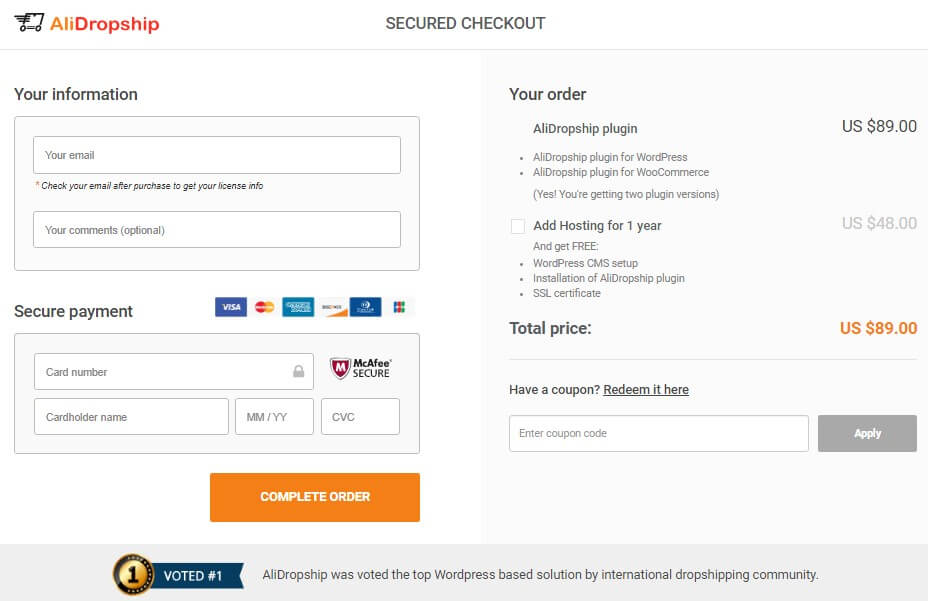This is a screenshot from the Allie Dropship secured checkout page. The Allie Dropship icon, which resembles a runaway shopping cart, features 'Allie' written in orange and 'Dropship' in red, combined into a single word.

On the left side of the page, there is a box for entering personal information including your email and comments. Below this box is the secure payment section, which requires the card number, cardholder name, card expiration date, and CVC. This section also displays logos of accepted payment methods, such as Visa, Mastercard, American Express, and Discover, along with a McAfee Secure logo, ensuring secure transactions.

On the right side of the page, order information is displayed. The order includes an Allie Dropship plugin for $89 USD. Bullet points highlight that the Allie Dropship plugin is compatible with both WordPress and WooCommerce. An option for ad hosting for one year is shown but is not selected, hence not included in the total price. The subtotal price of $89 USD is emphasized in orange.

There is a section to apply a coupon code with an 'Apply' button. Finally, an orange button labeled 'Complete Order' is prominently displayed for finalizing the purchase.

Additionally, the website boasts a recognition of being voted the number one WordPress-based solution by the international dropshipping community.